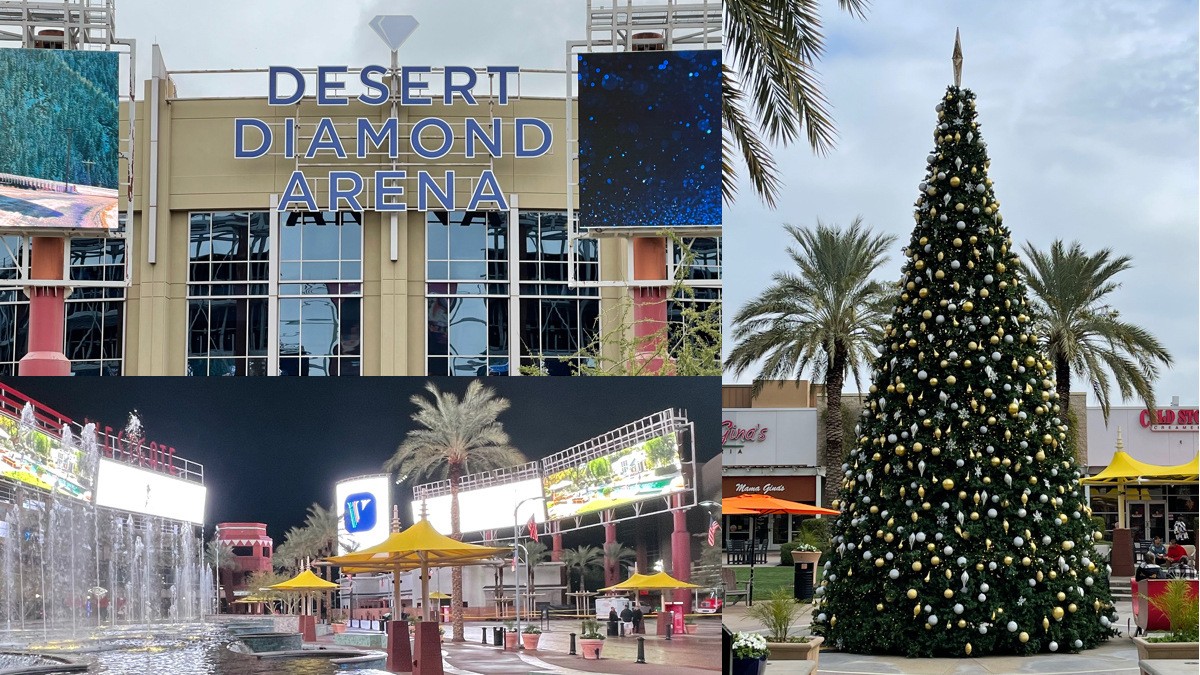The image is a detailed collage showcasing scenes from what appears to be a shopping center, likely in California, near the Desert Diamond Arena. The main focus on the right is a large, elaborately decorated artificial Christmas tree adorned with silver and gold ornaments, including bulbs of various shapes and a star at the top. Framing the tree are two palm trees, injecting a Palm Springs vibe into the scene despite the festive decorations. In the background, you can spot two businesses, one of which is Cold Stone Creamery, alongside outdoor seating areas equipped with vibrant orange and yellow umbrellas.

The upper left section of the collage is a close-up of a beige-colored building with numerous windows, marked by a sign that reads "Desert Diamond Arena." Flanking this building are electronic billboards mounted on tall orange poles. Beneath this image, in the lower left corner, is a nighttime view of the same area. Here, illuminated billboards, decorative water fountains, and the same distinctive umbrellas are visible, adding a lively glow to the palm-tree-lined outdoor space. This inset photo captures the dynamic ambiance of the location both during the day with clear blue skies and at night lit up with vibrant lights.